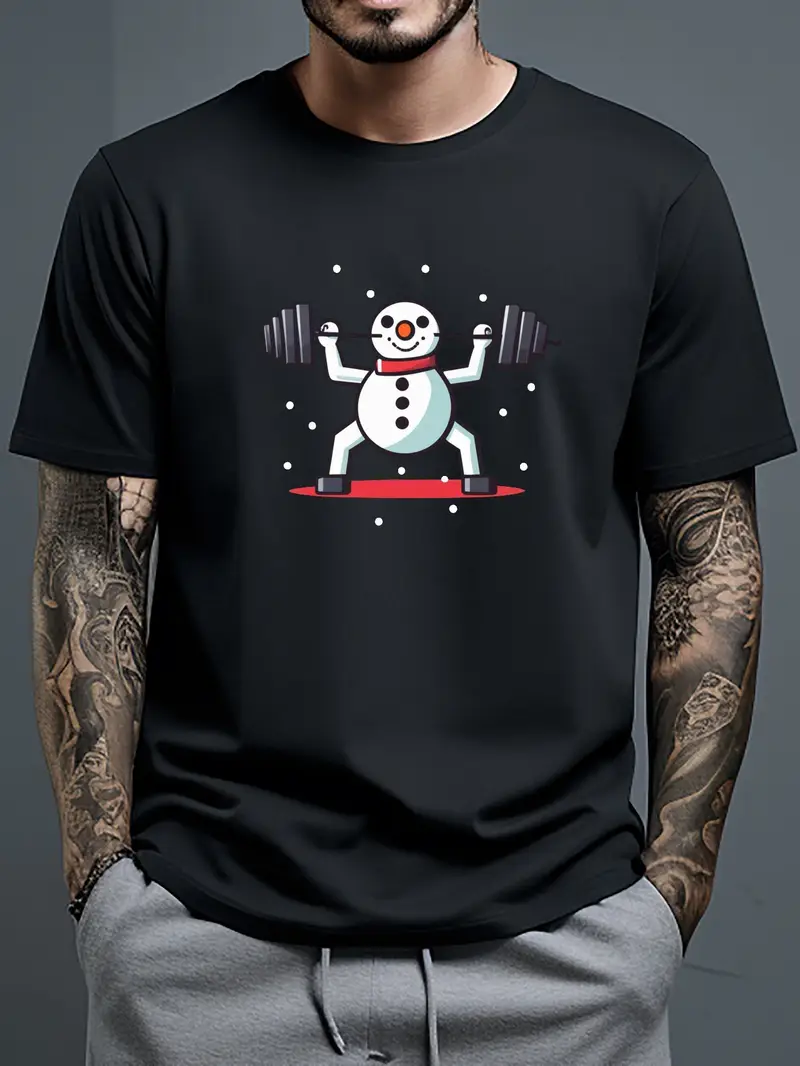In this image, we see a close-up of a man modeling a black T-shirt adorned with a festive snowman design. The snowman, depicted with beady eyes and an orange carrot nose, is wearing a red scarf and features three black buttons down its front. The snowman appears to be lifting a barbell at eye level, with each end of the barbell loaded with three or four weights. The man’s face is mostly out of the frame, but he sports a dark, stout beard. His arms, fully sleeved with detailed tattoos, extend down to his hands, which are tucked into the pockets of his gray sweatpants. The background is a neutral gray, and the man stands on a red platform speckled with white dots resembling snow.